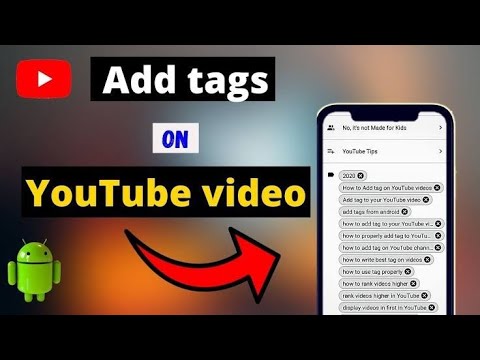This vibrant and colorful website features a sleek design with a minimalistic layout. At the top and bottom of the page, there are black horizontal bars providing a structured frame. Prominently displayed in the center is a red square with gently curved edges, containing a white arrow inside, labeled "Add Tags" in a bold, black box.

Below this, there is a white box with blue text stating "On" and the phrase "Your Tube Video" in a black box with yellow letters. 

In the top-left corner, an endearing green cartoon character with black eyes and antennae, made up of cylindrical shapes, catches the eye. Adjacent to this character is a red arrow, reminiscent of the Amazon logo's curve, directing attention towards an image of a smartphone screen. The smartphone displays the word "YouTube" and a phrase about content for kids, along with a list of various YouTube-related topics.

The website's background is a gradient of fading colors that seamlessly blend into each other, featuring shades of brown, red, orange, and white in the center, transitioning to darker grays around the edges, creating a striking and dynamic visual appeal.